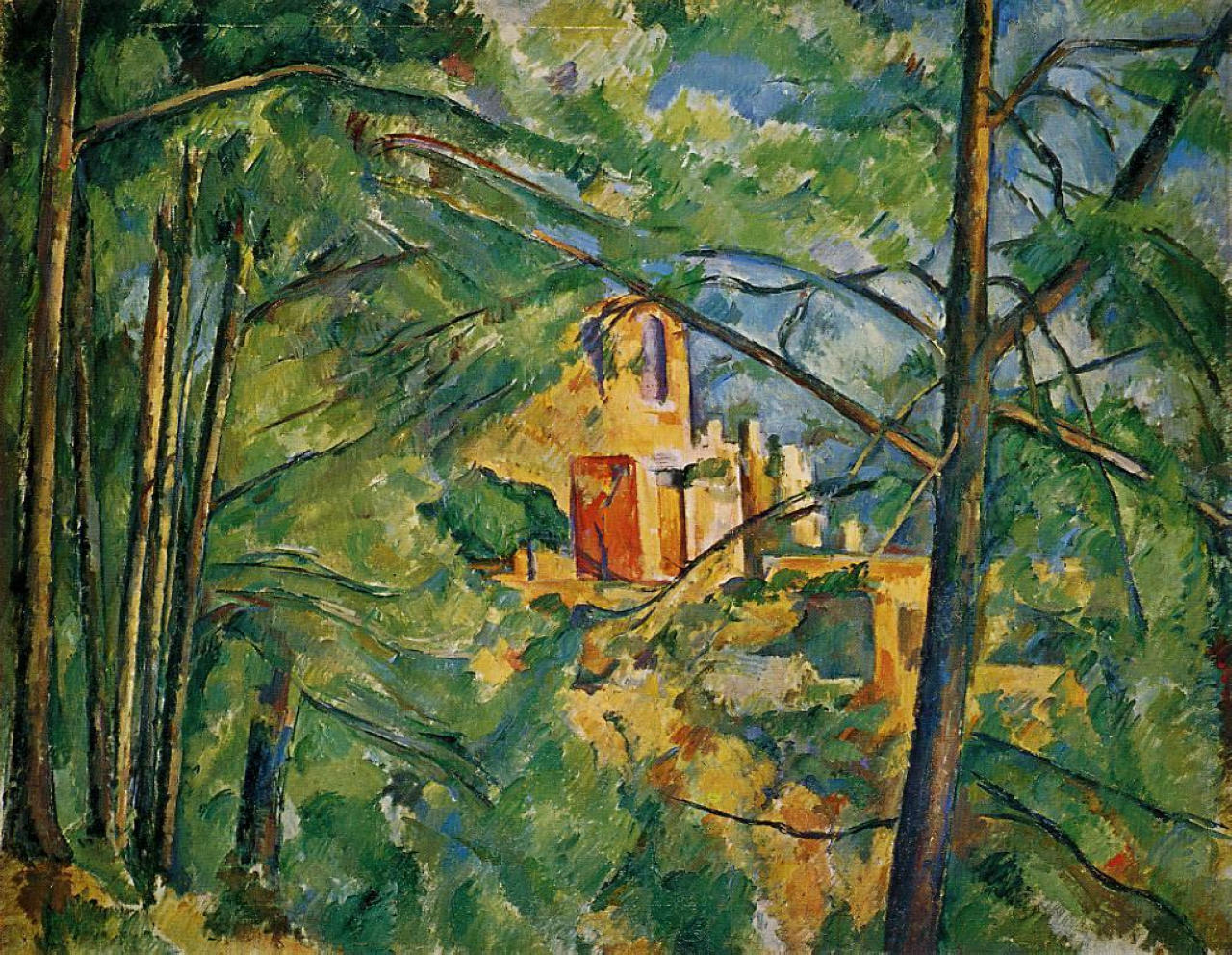This painting depicts a picturesque house nestled within a dense forest. On either side of the composition, tall, slender trees with green, leafy foliage rise up, punctuated by bold brushstrokes that suggest branches and leaves more than realistically portraying them. Through an opening between the trees, a mustard-yellow house with a reddish-orange door stands prominently in the middle, framed by a clear blue sky in the background. The house features dramatic black lines outlining its structure, adding a sense of depth and contrast. The entire scene is bathed in vibrant hues of green, yellow, and blue, with splashes of red subtly scattered throughout the painting, lending it a lively and dynamic feel. The use of bold brushstrokes and impressionistic techniques gives the artwork an old-world charm, while the details like white and yellow highlights add texture and light to the overall composition.